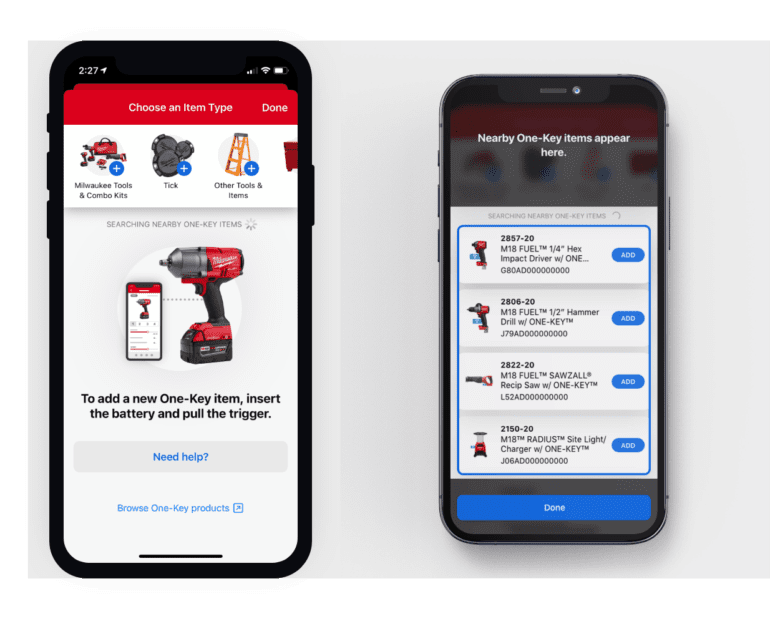Two iPhone screenshots are showcased against a grey background, with the left phone displaying a screen roughly two-thirds larger than that of the right phone. The left phone is set against a slightly lighter grey gradient. This larger smartphone shows a black outline, indicating its 2:27 p.m. time display in white numerals, along with the typical battery, Wi-Fi, and signal icons at the top right corner.

The highlighted content on the left phone is a website viewing a red Milwaukee drill. A prominent red banner at the top reads "Choose an item" with "Done" in white text. Below the product image, instructions say, "To add a new One-Key item, insert the battery and pull the trigger," followed by a "Need help?" button in blue text.

The right phone screen, slightly smaller in size, also features Milwaukee products but with a distinct blue background, suggesting it is from a different website.